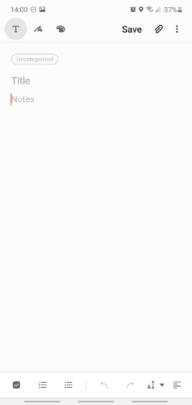The image is a screenshot depicting what appears to be a blank text entry or post creation interface. On the right side of the screen, there are several buttons: a prominent "Save" button, followed by a paper clip icon likely for attaching files. Below these, to the left, there is a greyed-out button labeled "Uncategorized." Further down, also in grey, is an area marked "Title," indicating where the user should enter a title for their post. Beneath that, there's a section labeled "Notes," with the cursor situated at the beginning of this field, ready for text input. At the very bottom of the screen, there are multiple options available for customizing text alignment, such as left, center, right, and possibly justify alignments, providing users flexibility in how their text will appear.